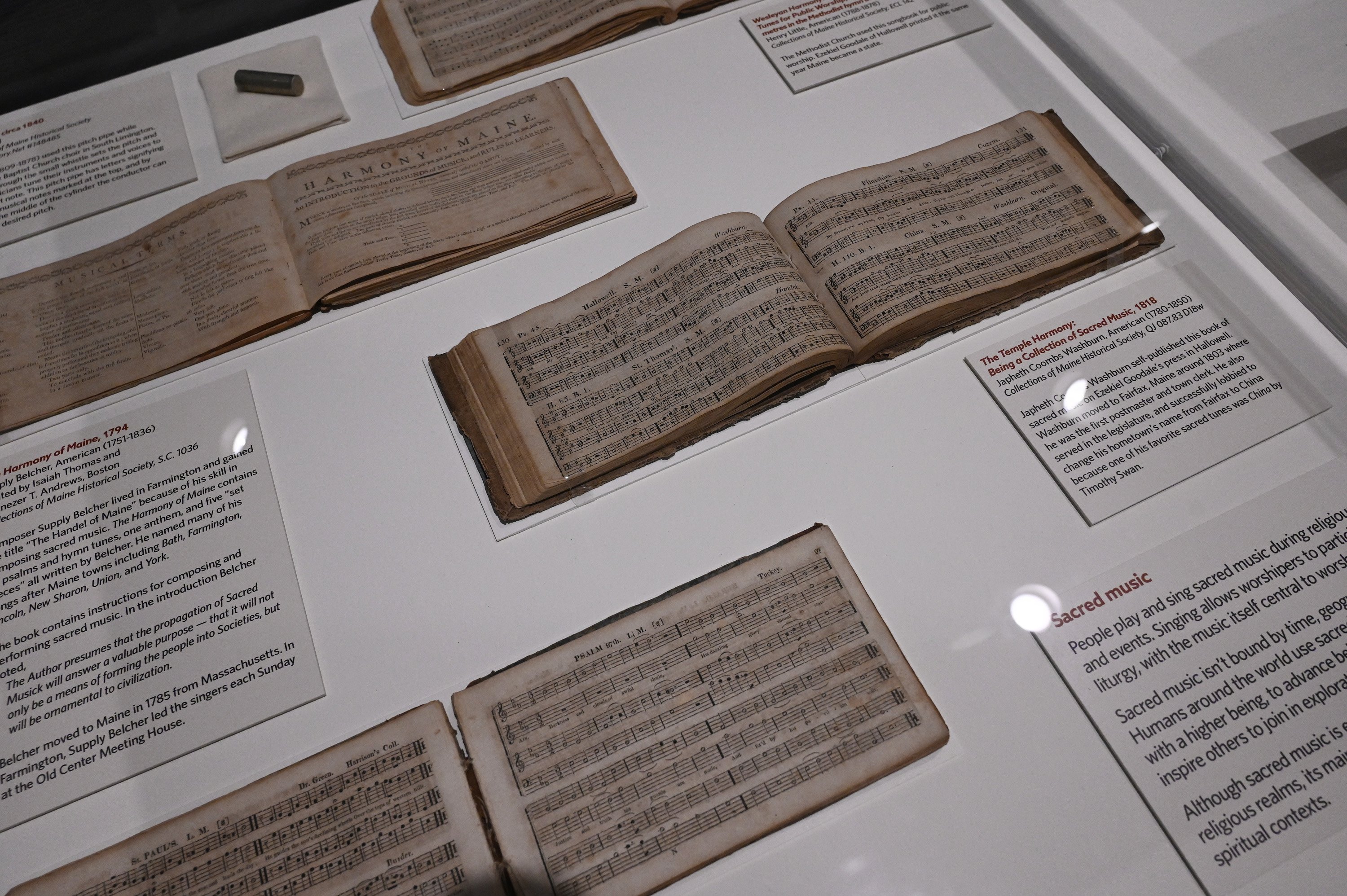This photograph appears to have been taken in a museum or a similar setting, showcasing a collection of old and possibly sacred sheet music books displayed through a glass case. The books are arranged on a large white surface, which could be a table or a wall. The books are positioned in an alternating pattern: one on the top right, one a little lower on the left, then another lower on the right, and one more lower on the left. They all lie open, revealing black musical notes on aged, brownish pages. 

Accompanying these books are white plaques featuring both red and black text. For instance, the plaque in the bottom right corner begins with 'Sacred Music' in red text and continues in black with an incomplete explanation about people playing and singing sacred music during religious events. These descriptive plaques provide details about the significance and historical context of each piece. 

The display is well-lit, with lights highlighting the books and the textual plaques. The overall setting and the informative plaques suggest these books are indeed sacred music pieces, offering a glimpse into their historical and religious importance.